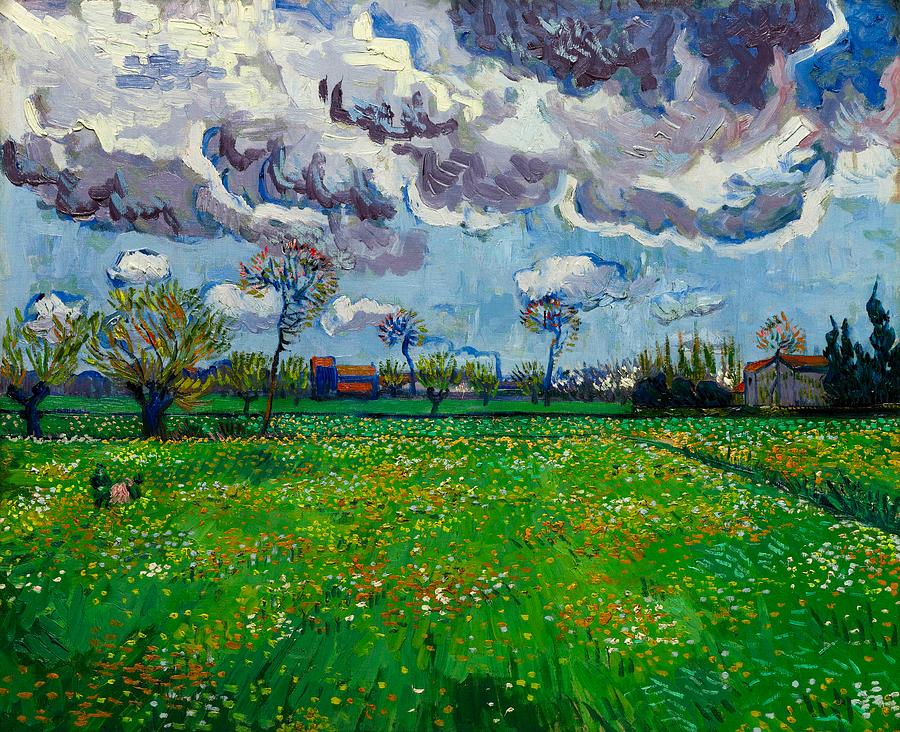The image is a detailed, textured oil painting, possibly by Van Gogh, featuring a vast field of multicolored wildflowers in shades of white, yellow, gold, and orange, set against a rich backdrop of greenery. The intricate brushstrokes give the painting a pointillistic feel, where tiny details collectively form a cohesive and aesthetically rich composition. In the distance, a row of stylized trees is visible, some with dark bluish trunks and leaves in hues of red, yellow, and green. Among them are tall, spirally cypress or cedar trees, iconic to Van Gogh’s style. There are also a couple of buildings, including a barn-like structure near these spirally trees. The sky, occupying nearly half the painting, is a dramatic expanse of ominous clouds, varying from harmless white to heavy, dark gray, suggesting an impending rainstorm, with patches of light and dark blue peeking through. There is also a small figure or couple on the left side of the meadow, adding an element of human presence to the natural landscape. In the far background, an industrial smokestack emitting blue smoke adds a subtle modern touch to this otherwise pastoral scene.